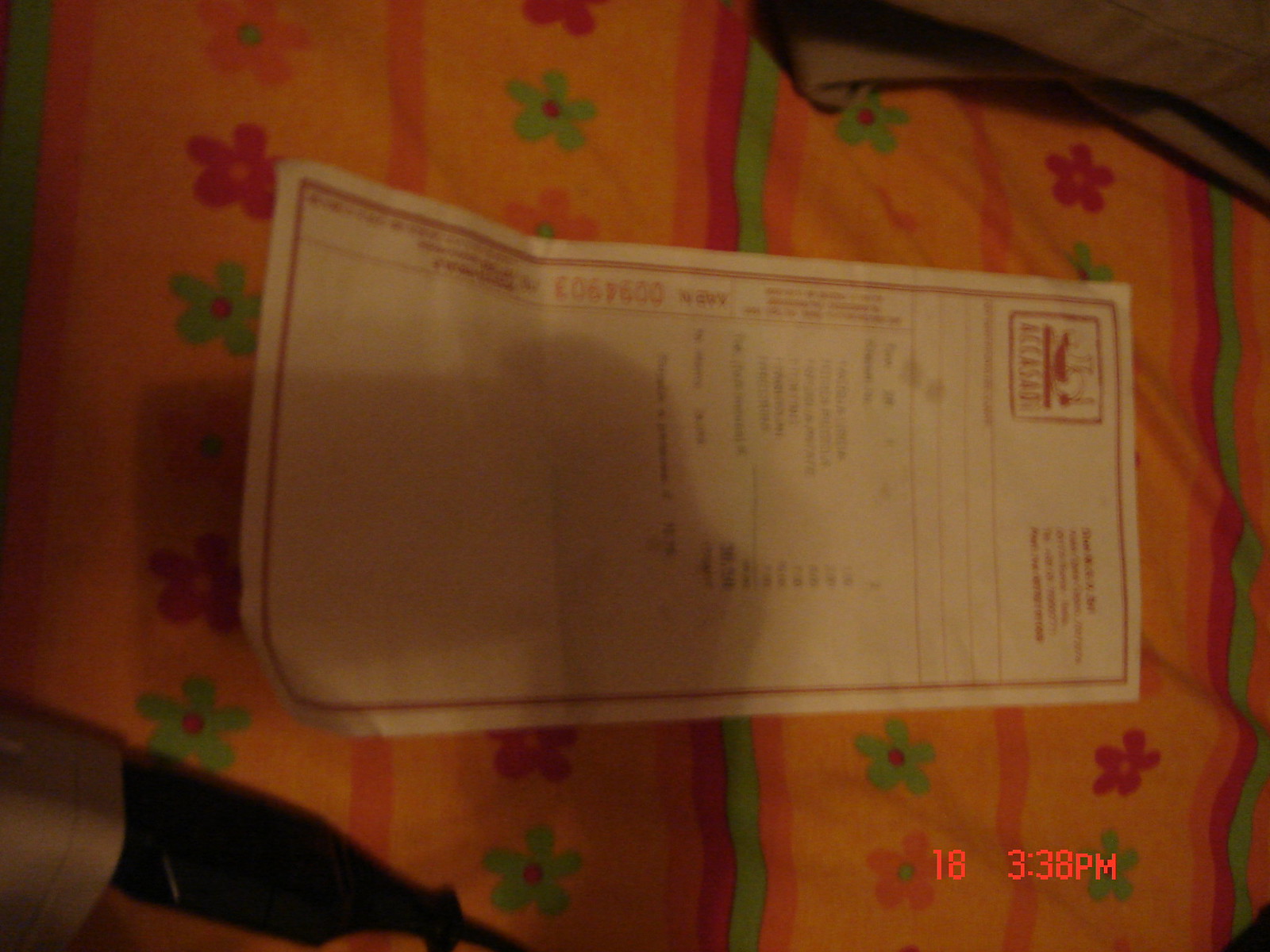A very blurry color photograph depicts a white piece of paper, possibly a receipt, lying on an orange cloth adorned with a floral pattern featuring red and green flowers. The paper is so indistinct that its contents are unreadable, though it seems to have red writing at the top and typed black text in the middle. A time stamp in the bottom right corner reads "18, 3.38 p.m." Beyond the timestamp, no legible writing is visible. The image is devoid of people, animals, plants, or buildings, solely focusing on the unclear document atop the vibrantly designed fabric.